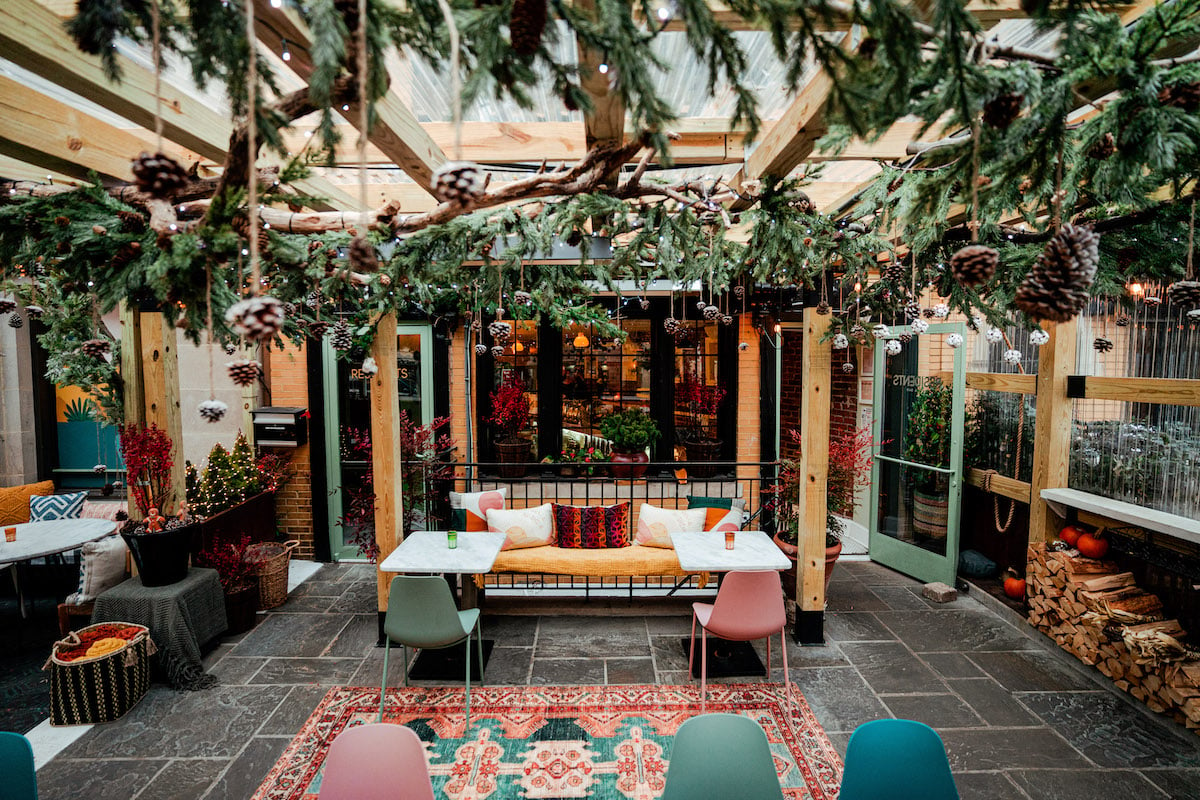This image depicts a stylish courtyard, likely part of a high-end restaurant or boutique hotel, that seamlessly blends indoor and outdoor elements. The space is partially covered by a translucent roof supported by wooden beams and columns, giving it a cozy yet open ambiance. The ceiling is adorned with boughs of evergreen and hanging pine cones, enhancing its natural charm. This courtyard is lavishly decorated with plush seating, including a prominent couch with pillows and cushions in shades of red, and a mix of colorful chairs, including pink and gray ones. A Turkish rug lies atop the black tiled floor, adding to the chic aesthetic. The setting is well-lit, with numerous plants cascading from the ceiling, creating a verdant canopy. On one side, there is neatly stacked firewood, adding a rustic touch. The space features several glass doors and large windows that provide views into a posh, colorful interior dining area. Though it evokes the tranquility of an outdoor setting, the abundance of windows, lights, and greenery makes it feel like a luxurious indoor atrium.